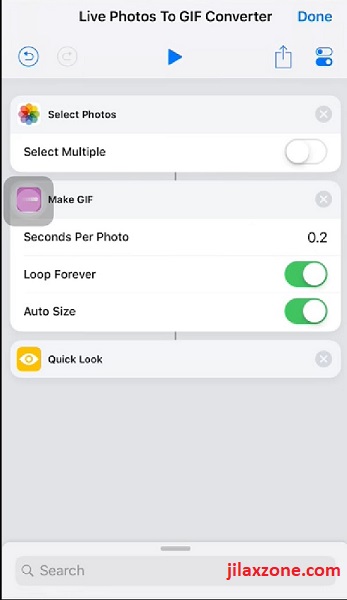This screenshot captures an interface from a software application named "Live Photos to GIF Converter," set against a light gray background. The title, "Live Photos to GIF Converter," is prominently displayed at the top. In the top-right corner, there's a "Done" button for completing the current task. Below this, the toolbar features buttons for "Undo," "Play," "Download," and two toggle options.

Moving further down, there are options labeled "Select Photos," "Select Multiple" (currently toggled off), "Make GIF," and "Seconds per photo: 0.2." Both "Loop Forever" and "Auto Size" options are toggled on, indicating that the GIF will continuously loop and automatically adjust its size.

A gray oval button labeled "Quick Look" is also present, featuring a yellow square icon with a white eyeball, suggesting a preview function. The rest of the interface continues in the same light gray background. At the bottom of the screen is a gray bar containing a search bar. In the bottom-right corner, the URL "JILAXZONE.com" is displayed in red text.